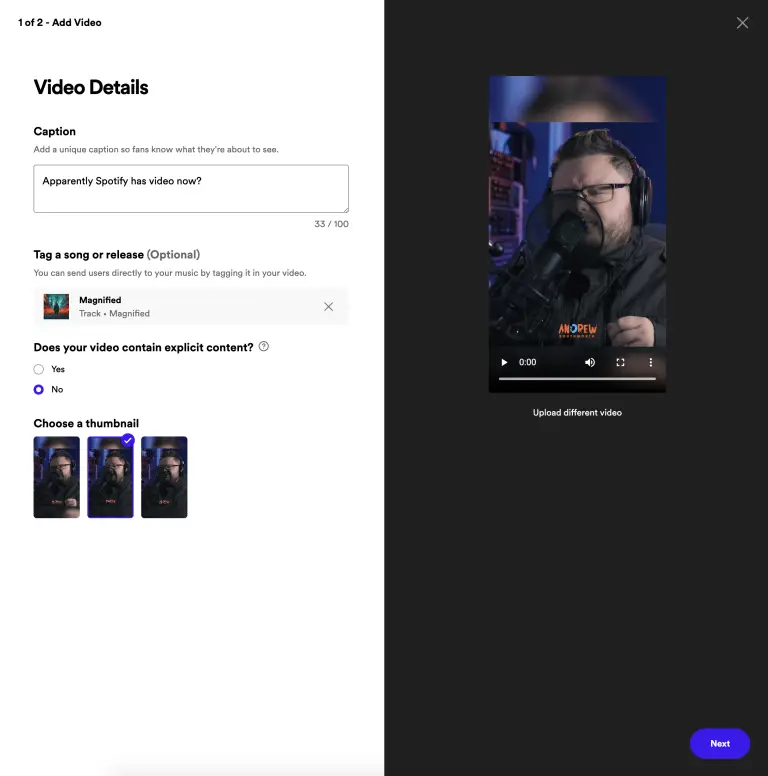The image depicts a web page interface designed for uploading videos. The top left corner features the text "1 of 2 - Add Video" in black font against a white background. Directly below it, in a larger black font, is the heading "Video Details." 

Under this heading, a sub-section labeled "Caption" instructs users to "Add a unique caption so fans know what they're about to see." A text box is available for inputting these details, and an example caption reads, "Apparently Spotify has video now."

Following the caption section, there's an option to "Tag a Song or Release," marked as optional. In this example, the user has tagged a track named "Magnified," with an adjacent 'X' icon allowing for the removal of the tag.

The next section asks, "Does your video contain explicit content?" The radio button next to "No" is selected, indicating the video does not have explicit material. Further down, there's an option to choose a thumbnail for the video.

On the right side of the screen, set against a black background, is a preview of the uploaded video with a play button overlay. Below the preview, a link labeled "Upload different video" is provided, offering the user an option to select an alternative video for upload.